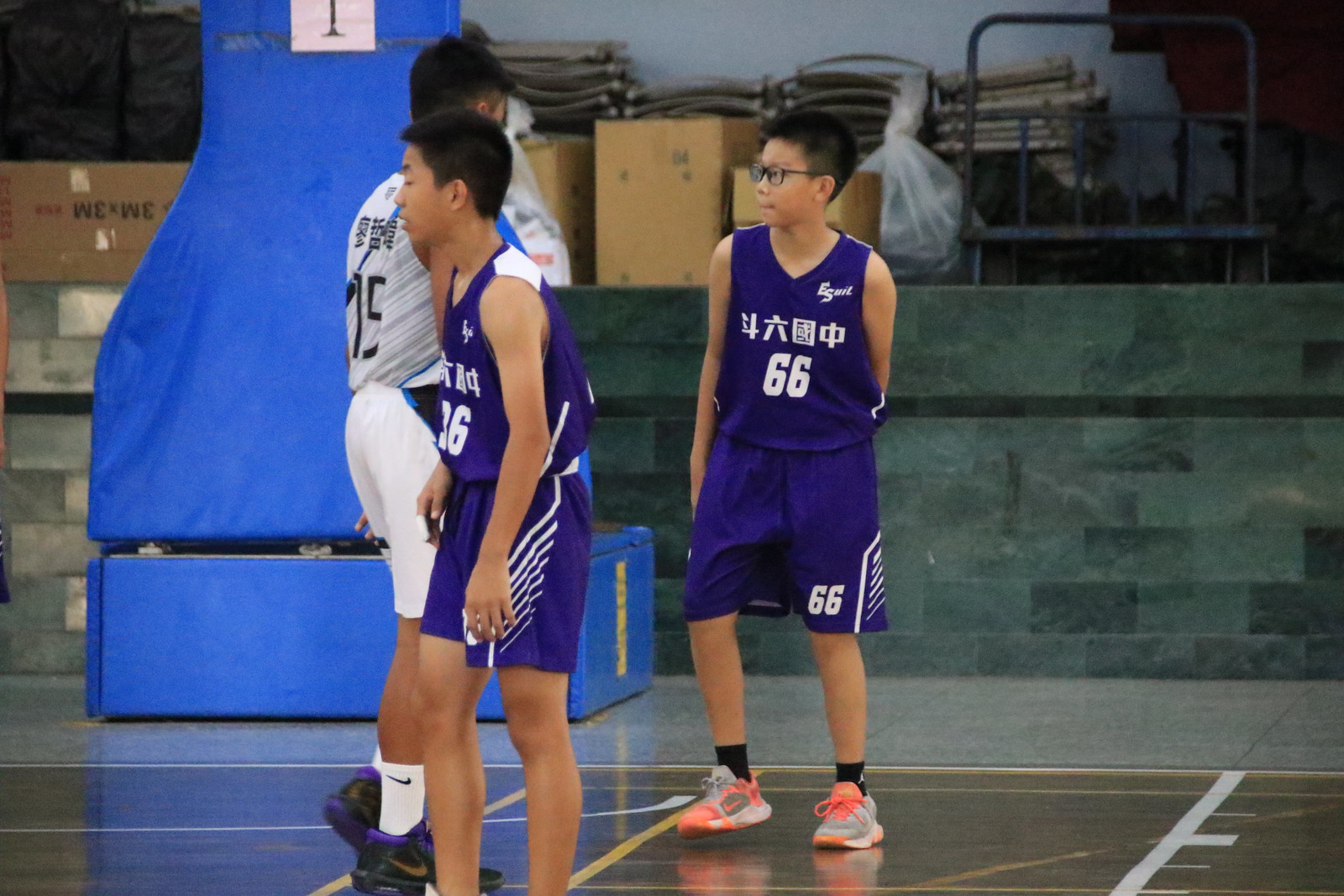The image depicts an indoor basketball scene, likely set in a gymnasium with a shiny, non-wooden floor. In the foreground, there are two teenage boys wearing deep purple basketball uniforms, adorned with Japanese or Chinese characters. Both teens have buzz cuts; the boy wearing jersey number 66 has black-framed glasses and is sporting gray and pink sneakers, while his teammate in jersey number 36 does not wear glasses. They appear to be around 13 or 14 years old. Both are standing underneath a blue-padded basketball hoop holder, facing right to left as if observing something off-court. Positioned between them is a taller individual in a predominantly white referee uniform, numbered 15, seen from behind. This referee is dressed in white shorts paired with black tennis shoes and appears to be walking in the opposite direction. The scene captures a moment of pause, possibly during a timeout, as the players are not actively engaged in play.